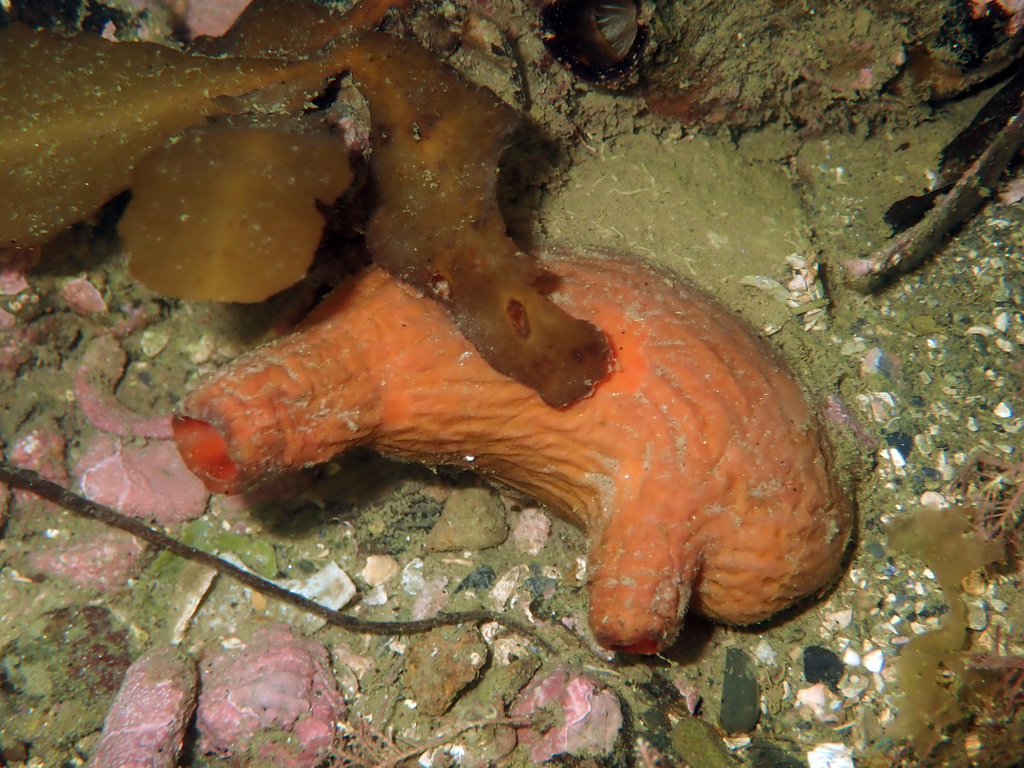This underwater image showcases a fascinating scene on the seafloor featuring a prominent, large tubular orange organism that appears wrinkly and pruned. Resembling an orange organ with a shriveled appearance, it has an open tube at one end and another tube-like structure near the bottom side that may be closed off. The organism is surrounded by a mixture of greenish-brown sand, scattered white shell fragments, and several pink stones or corals. To the upper left of the organism, drooped above, there is a leaf-like, seaweed structure with yellowish-brown accents. The seafloor itself is speckled with various small, glass-like objects of different colors including purple, green, red, and possibly black, adding to the intricate and colorful composition of the scene.